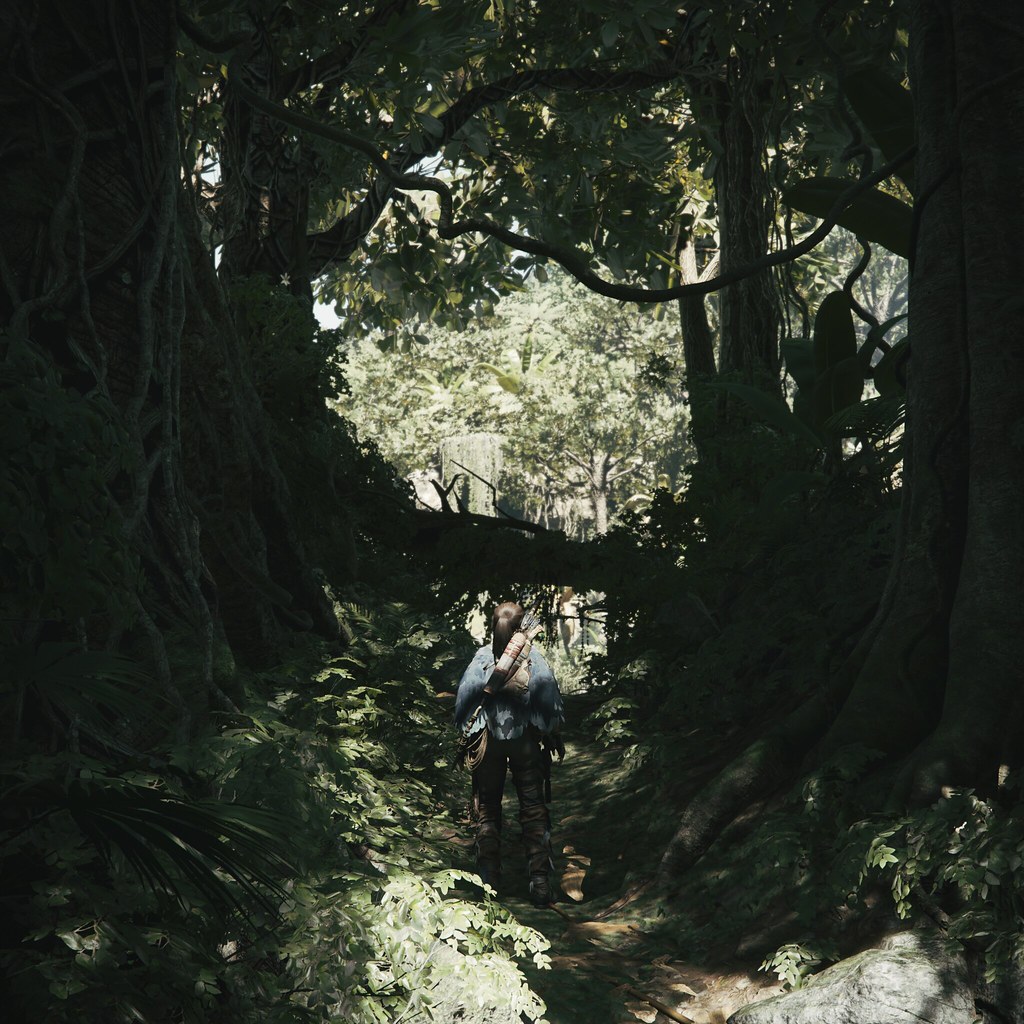A photograph captures a serene nature scene on a sunny day, featuring a dry creek bed flanked by towering trees, resembling cypress with thick trunks and abundant greenery. In the center, a woman, possibly a hiker, stands with brown hair tied in a ponytail. She wears a denim jacket, jeans or pants, and hiking boots, with a backpack and possibly some gear slung over her shoulder. The scene is shaded by the dense canopy overhead, with exposed roots and thick vines covering the ground around her. Ahead, a trail winds upward, flanked by more dense foliage, rocks, and a fallen log stretching across the path. Bright sunlight filters through the trees beyond, highlighting the lush greenery and creating a stark contrast between the shaded area where the woman stands and the sunlit background.